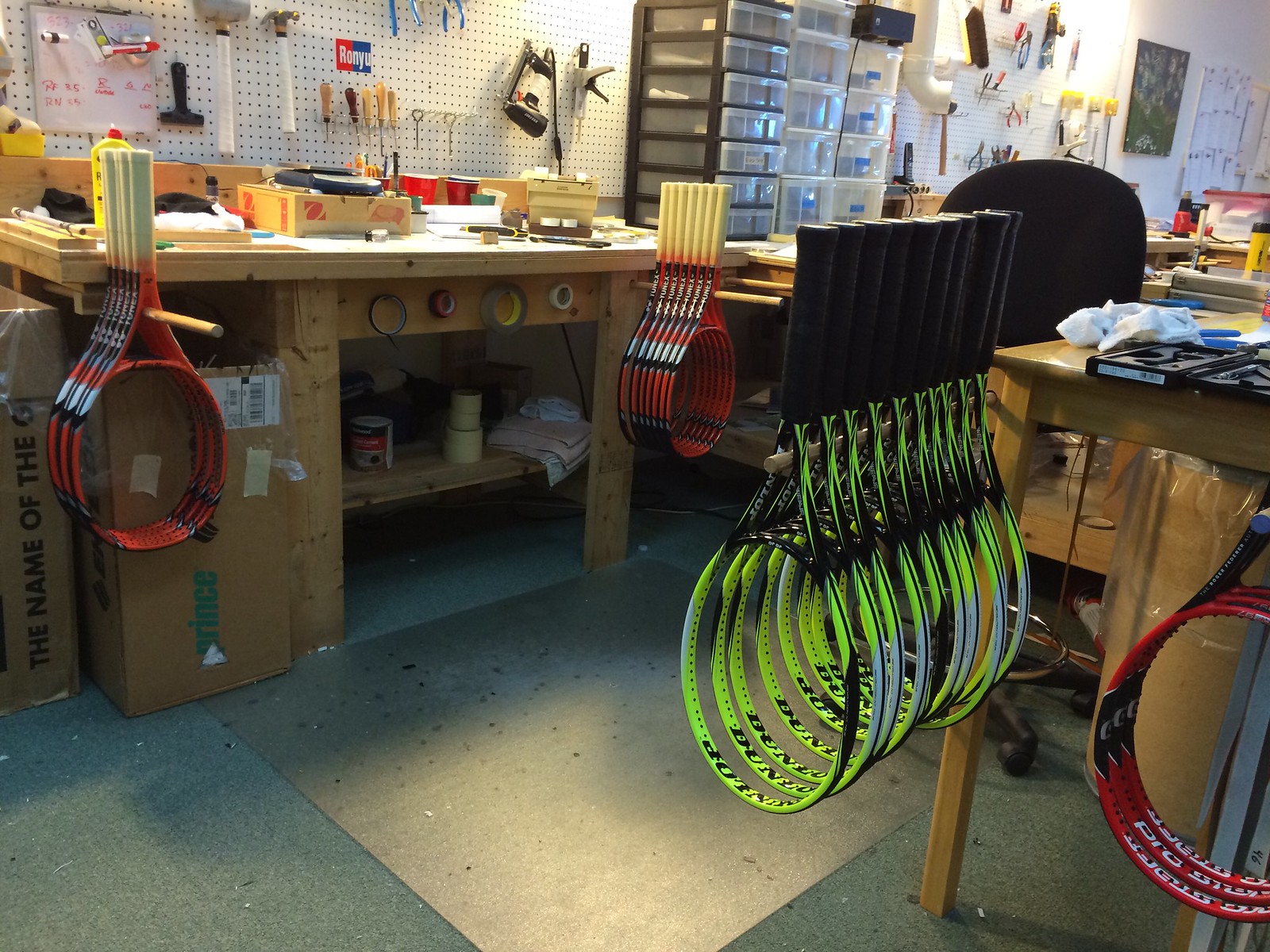The image depicts a detailed view of a tennis racket workshop. Dominating the foreground are multiple wooden workbenches, two of which occupy the left and right sides of the image. Each workbench features wooden dowels on which tennis rackets are hung through their handles, with their heads facing downward. These rackets are organized in rows; the left side predominantly displays red rackets with white handles and black accents, while the right side showcases a variety of rackets, including red and fluorescent yellow-green ones. The yellow-green rackets have black grip handles and the name "Dunlop" printed on them. There are approximately 15 to 20 tennis rackets in total, many of which lack netting or strings as they are in the process of being completed.

Further details reveal additional elements of the workshop: on the left, behind the workbench, is a white pegboard filled with various tools such as hammers and vices, as well as a small whiteboard with markers. Below this workbench, two boxes sit on the dark green carpeted floor. The far background on the left side features tall plastic shelves and another pegboard holding more tools. There is a black chair visible towards the back, complementing the organized chaos of the workspace. This workshop environment, replete with hanging tools, plastic bins, and containers, and light-colored wooden workbenches, appears to be set up for the meticulous task of stringing and preparing tennis rackets.